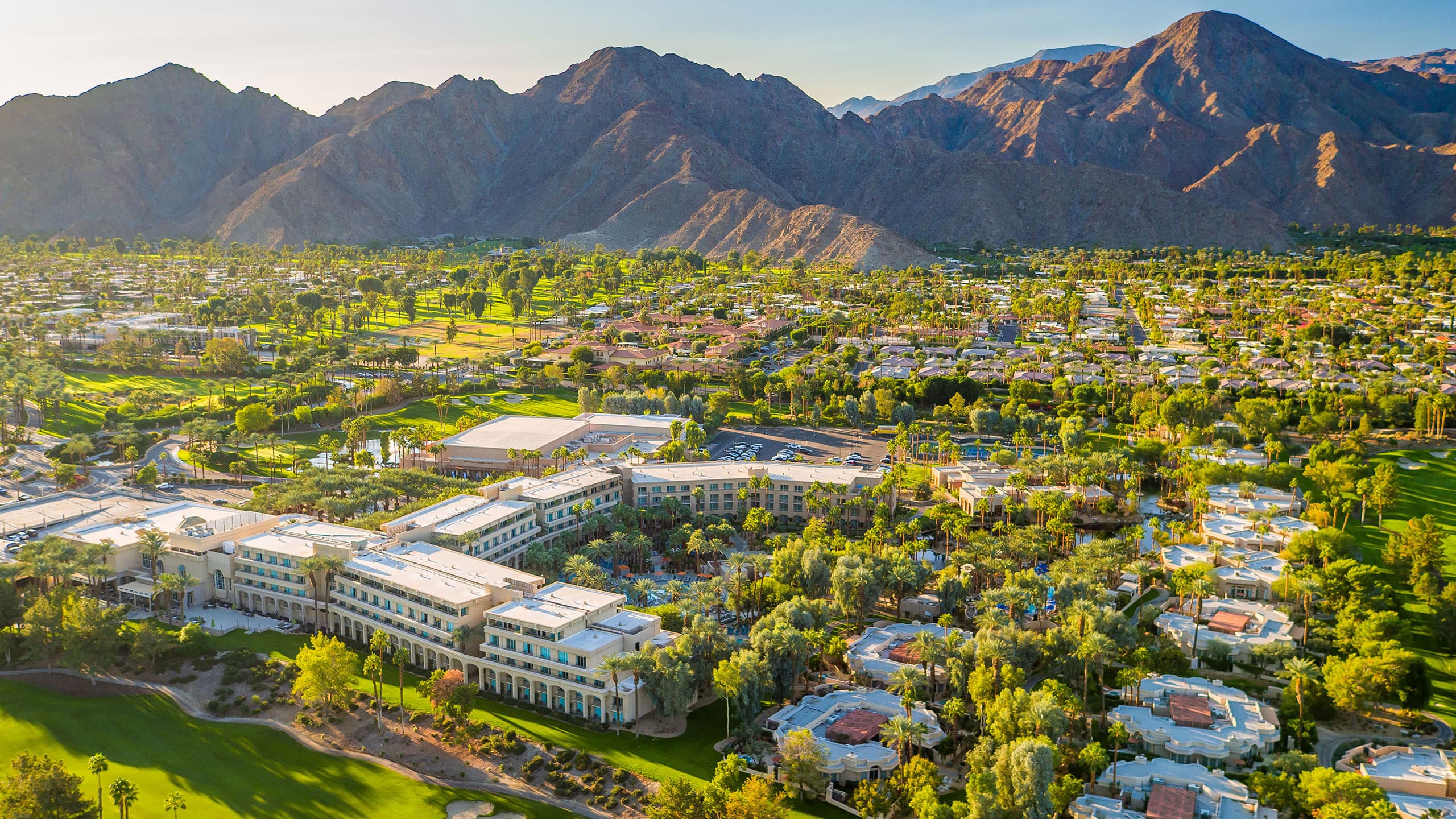This aerial photograph captures a scenic valley enclosed by a range of tall, rocky mountains that span the entire top third of the image from left to right under a clear blue sky. The mountains, devoid of snow, form a stark, brown backdrop to the vibrant scene below. The lower two-thirds of the image showcase a lively town set amidst lush greenery. The landscape is peppered with regular trees typical of California, adding to the verdant and vibrant atmosphere. The center of the town is dominated by numerous buildings with white roofs, luxurious condos, pools, and scattered vehicles. On the right side of the foreground, we see several circular structures organized in neat columns and surrounded by trees. Towards the bottom left corner, there is a golf course with well-manicured green grass and a sand dune. The middle section features rows of four-story buildings with numerous windows, while suburban homes with red roofs and white walls are visible further on. The image conveys the allure of a potential vacation destination brimming with life and activity.